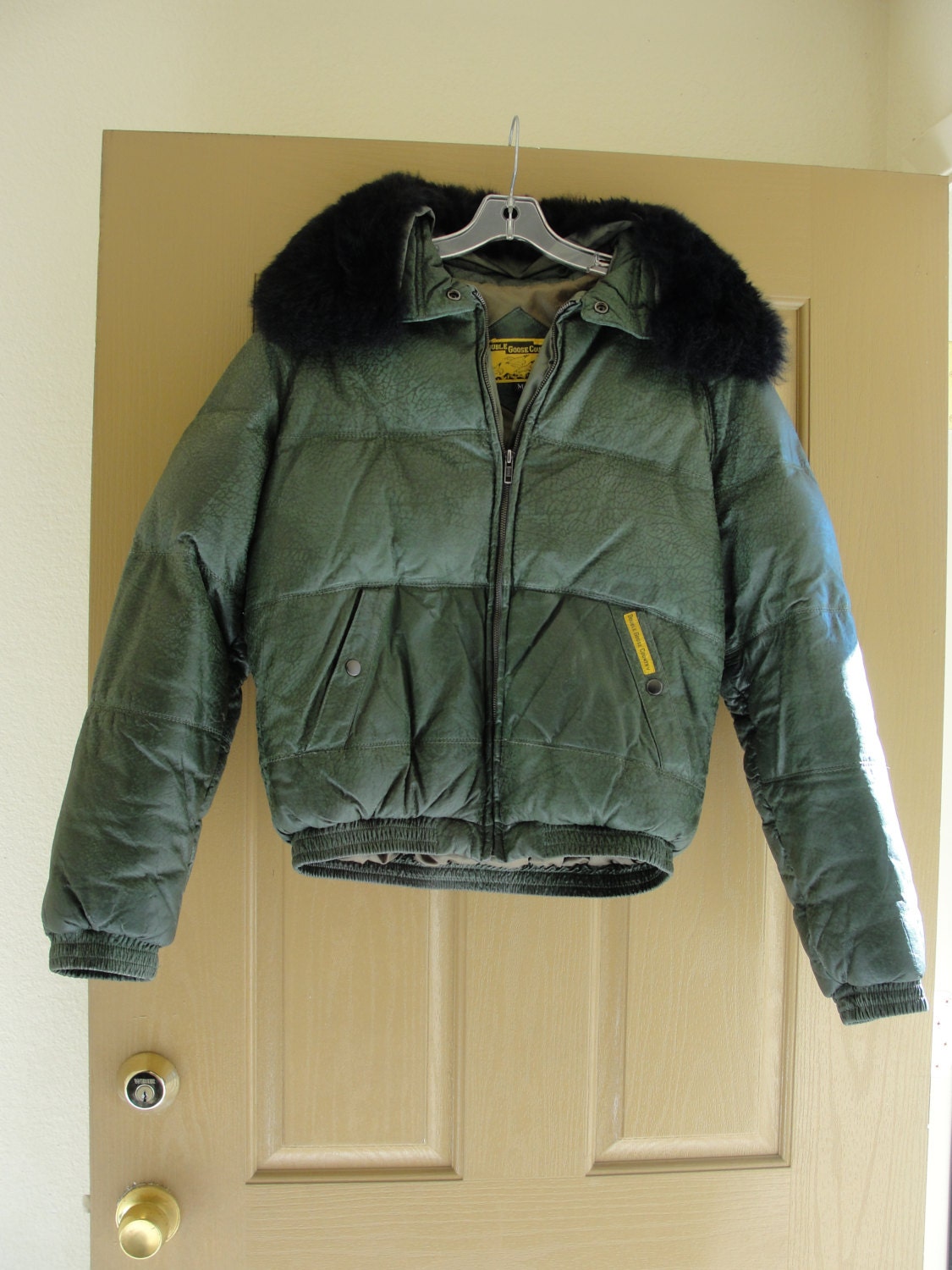This photograph features an army green puffer jacket designed for winter, prominently displayed hanging from a light tan wooden door. The door, adorned with a shiny gold doorknob and deadbolt, contrasts with the off-white wall behind it. The jacket boasts a black fur or faux fur-trimmed hood, adding a cozy element to the thick, insulated design. The jacket’s sleeves and bottom are elasticized for a snug fit. Visible details include a small, indistinguishable yellow patch on one of the front pockets and a similarly indiscernible yellow label inside the back neck area. The two front pockets are diagonal slit style with snap closures, adding to the functional and stylish appearance of the garment. This image might be used for online marketplaces like eBay or Mercari, aiming to showcase the jacket's features comprehensively.